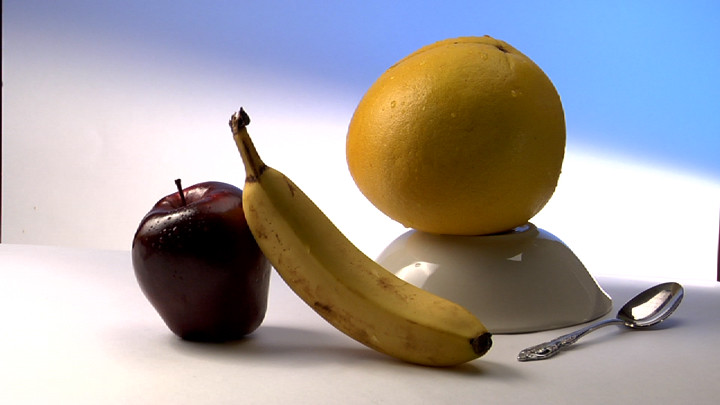A meticulously arranged fruit display is set against a distinct, blurred background of blue and white light. At the center, an upside-down cereal bowl sits prominently, with a gleaming lemon perched firmly on top, showcasing its fresh, uncut exterior. Beside the bowl lies a simple spoon, hinting at a minimalist yet intentional placement. Flanking the setup, there is a dark red apple, standing upright with its stem intact and looking freshly picked. Nestled next to it is a perfectly ripe banana, leaning against the apple for support, indicating it's at the peak of its ripeness. The ensemble rests on a pristine white surface, likely a table, lending a clean and uncluttered aesthetic. Subtle reflections dance in the bowl, adding a touch of visual interest and highlighting the careful composition of the scene.